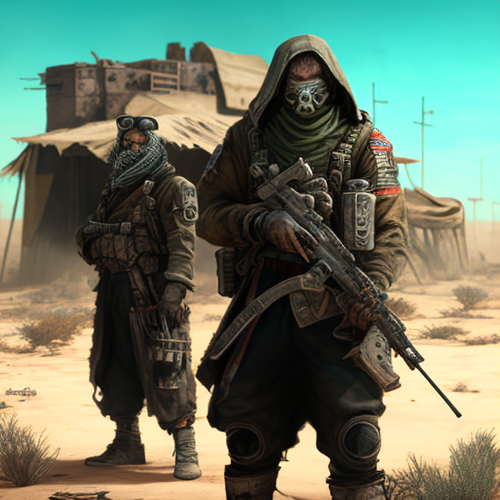This detailed CGI or AI-generated illustration depicts two heavily dressed mercenaries or soldiers in a desert or post-apocalyptic setting. Both figures are shrouded in weathered tan clothing, adorned with various utility straps and gear. The individual in the foreground is especially prominent; he wears a green hood, a full-face mask with only his eyes and part of his forehead visible beneath the hat, and a gray infinity scarf. Additional details include a red, blue, and white shoulder patch, gloves, knee pads, and nearly knee-high boots. He holds an AR-style assault rifle with an extended barrel. The second figure in the background mirrors a similar rugged attire, featuring a shawl-like headscarf and boots, and stands near a crude structure, all set against a backdrop of desert flora and distant buildings. Their stern gazes and imposing presence add to the menacing atmosphere of the scene.